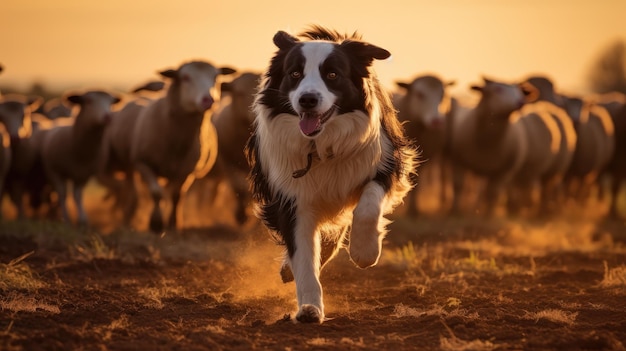In this image, a happy border collie runs energetically towards the camera, leading a flock of sheep down a dusty, dirt path. The black and white dog, identifiable by its white chest, paws, and a distinctive white stripe running from its nose up to its forehead, is in clear focus, tongue out in mid-trot, with its front left paw raised and other paws slightly off the ground. The background is filled with a multitude of white-faced sheep covered in grayish fleece, all slightly blurred to emphasize the motion. The entire scene is bathed in the soft, sepia tones of early morning or late afternoon light, giving the image a warm, nostalgic feel. The dusty path beneath the dog's feet further accentuates the dynamic movement, as small clouds of dust rise behind it. The scene captures a quintessential moment of pastoral life, with the diligent sheepdog joyfully guiding its flock.